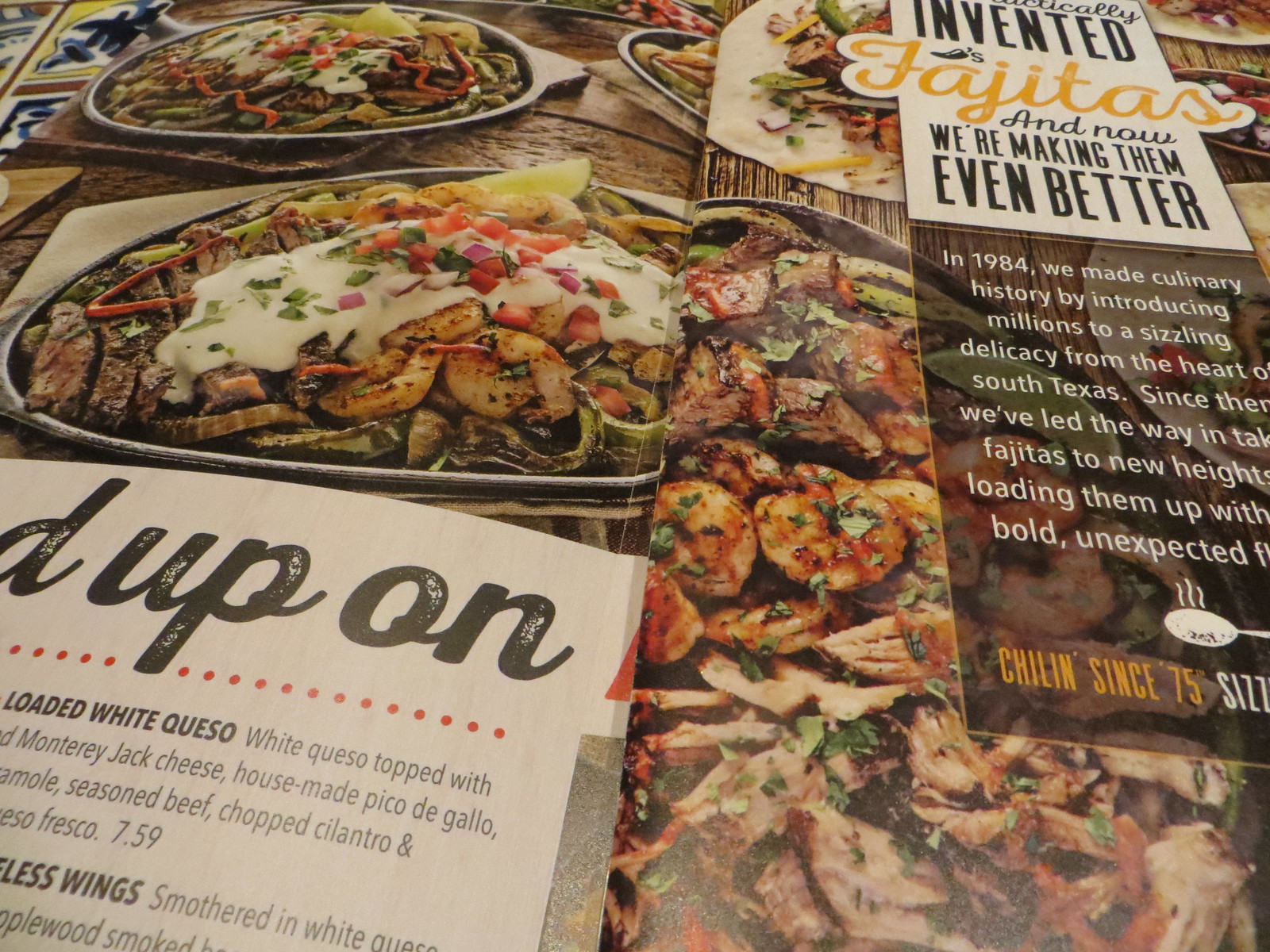The image depicts a vibrant menu or magazine page from Chili's showcasing a variety of inventive fajitas, emphasizing their culinary significance since 1984 when Chili's introduced them as a sizzling delicacy from South Texas. The text, "Invented Fajitas" and "Now We're Making Them Even Better," highlights their continued innovation with bold, unexpected flavors. The fajitas are presented with ingredients such as shrimp, chicken, steak, onions, peppers, and white queso, all vividly arranged on metal plates. Accents include house-made pico de gallo, guacamole, cilantro, and Monterey Jack cheese. The rich visual detail and nostalgic text underscore Chili's legacy with the tagline, "Chilin’ Since '75."